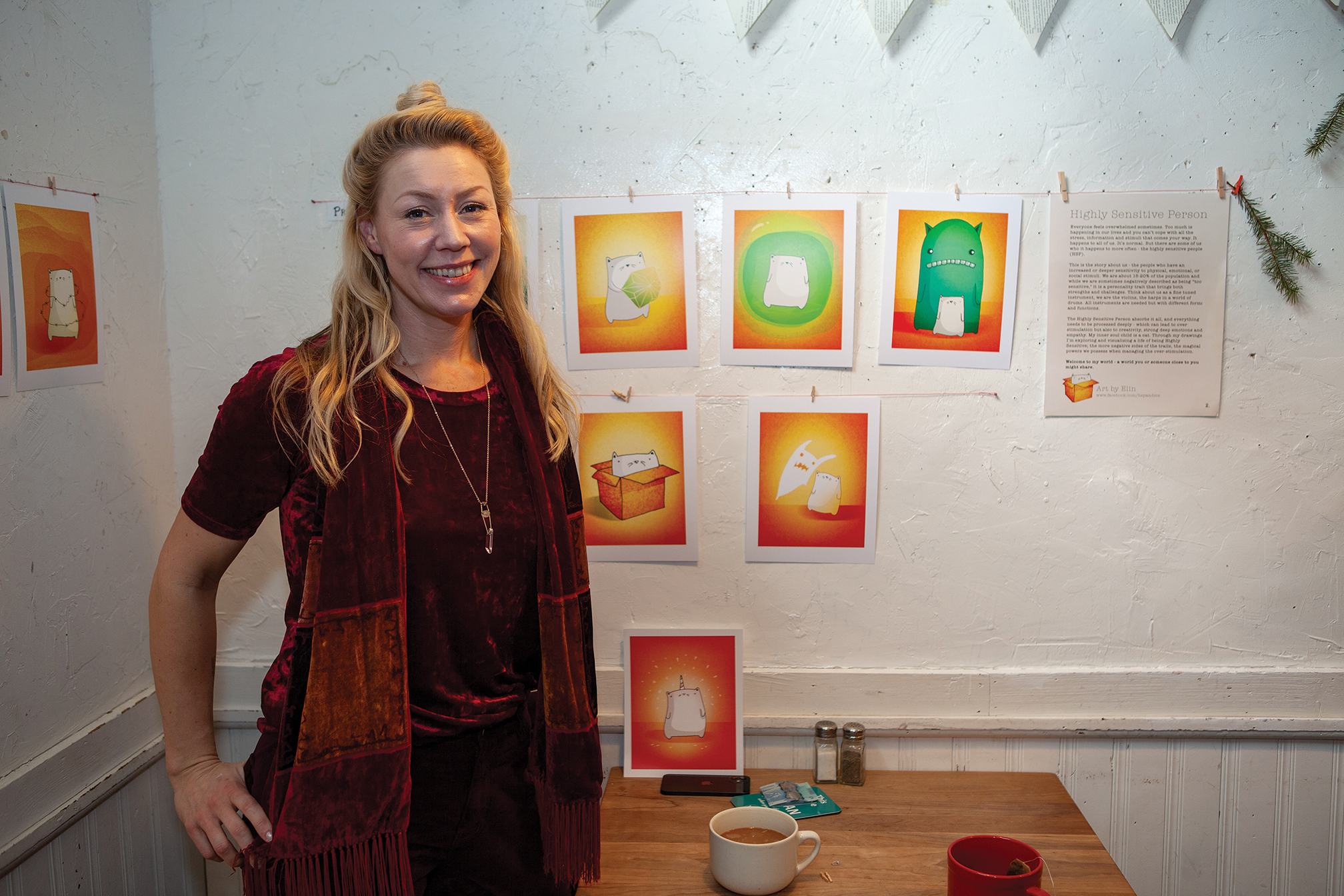In this vibrant color photograph, a cheerful female artist stands slightly left of center, proudly displaying her collection of animated artwork. She has long blonde hair, which she wears in a half-up bun, and she is dressed in a dark reddish-brown velvet dress adorned with a distinctive pendant necklace. Behind her, on a pale grey wall, are five pieces of her artwork, each characterized by an orange background and featuring various whimsical critters. These characters—a mix of cat-like creatures, green monsters, and hybrid catacorns—illustrate different emotions and sensitivities, with one piece showing a character wrapped in barbed wire. The images are clipped to lines with clothespins, alongside an artist statement and a "Highly Sensitive Person" sign.

On a light brown wooden table in front of and behind the artist, there are various objects, including two mugs of coffee (one white and one red with a tea bag), a green card, a salt and pepper shaker, and what appears to be a cell phone. A framed piece of her artwork also rests on the table, next to a few sprigs of pine used as decoration. The entire scene is suffused with the warm tones of her art and showcases the artist's evident pride and joy in her creations.